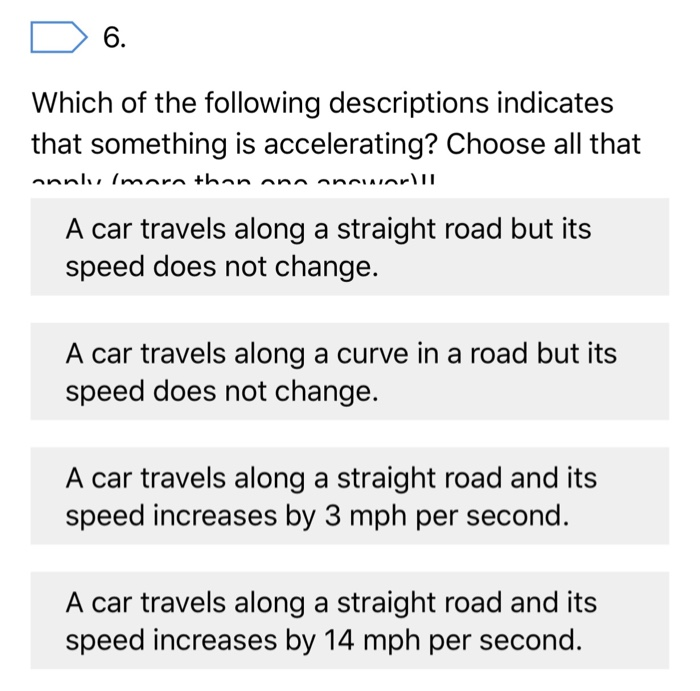Screenshot Description: 

The screenshot appears to be a question from a quiz or test. At the top left corner, there is a shape resembling a rectangle, but with the right side extending into what looks like the end of a triangle, suggesting it might be a hexagon. This shape has a blue outline. To the right of the shape, the text "6." is displayed, indicating the question number. The row is otherwise empty.

Below this, there is a line break, followed by the quiz question, which reads: "Which of the following descriptions indicates that something is accelerating? Choose all that apply." However, the instructions for selecting the answers are partly obscured by the answer choices, making them only partially readable—suggesting it might continue with "answer" enclosed in parentheses and possibly some punctuation.

The answer choices are presented in a white box that overlaps and partially blocks the question text. Within this box are four light gray selection boxes, each with black text. The options are:

1. "A car travels along a straight road, but its speed does not change."
2. "A car travels along a curve in a road, but its speed does not change."
3. "A car travels along a straight road and its speed increases by 3 MPH per second."
4. "A car travels along a straight road and its speed increases by 14 MPH per second."

This detailed description captures not only the visual elements but also the structure and partial layout issues indicated in the screenshot.